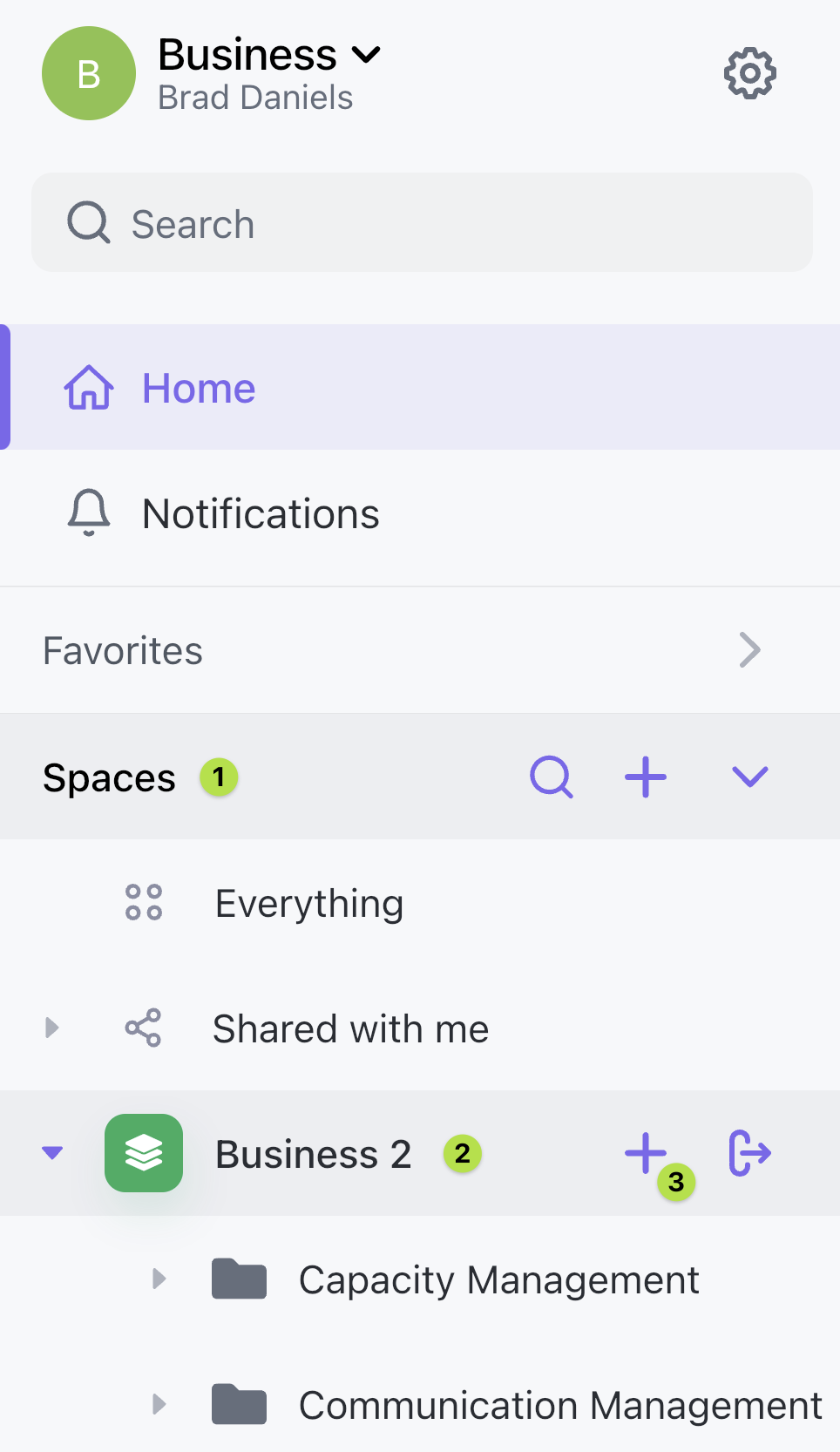The screenshot is from a mobile application featuring a "Business" tab at the top with a down arrow beside it. Directly beneath this is a header reading "Brad Daniels" with an avatar on the left—a lime green circle with the initials "ME" inscribed—and a gear icon on the far right. Below this header is a search bar, followed by navigation icons: a highlighted home icon, a notifications bell, and a favorite section. A "Spaces" section is also present with a lime green circled number one. Additionally, there is a magnifying glass icon, a plus button, and a down button. Under the "Spaces" section, two categories are listed: "Everything" and "Shared with Me." The "Business" category branches into "Capacity Management" and "Communication Management," each depicted with manila folder icons. The overarching "Business" category itself is represented by icons of stacked papers on a green background.